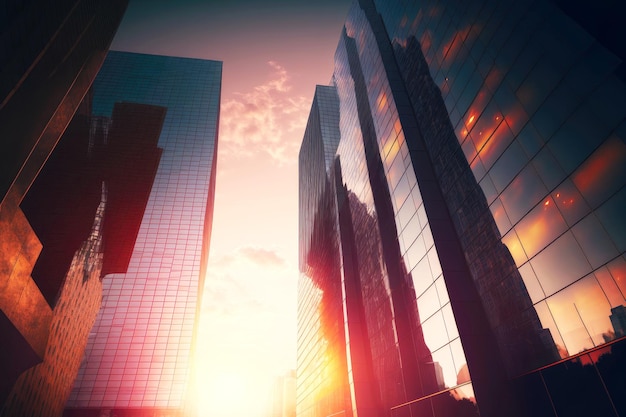This image features a rendered cityscape viewed from below, capturing a series of mid-sized skyscrapers in an enchanting moment as the Sun rises between them from the center-left. The sunlight bathes the buildings in red hues, accentuating the detailed architecture. The scene consists of three buildings on the right with a gap where the Sun's brilliant light peeks through, and two buildings on the left. One of these left-side buildings, which seems to be constructed of glass, reflects a distorted image of another structure. The sky above the rising Sun transitions from a dirty red to a pure yellow near the bottom center, with light pink hues and scattered clouds framing the skyline. Windows speckle the buildings, some warmly lit from within. The rightmost building boasts a sleek, dark glass facade, while the left side includes a white structure with a square pattern and another that appears orange or brick-like. The cityscape hints at a bustling urban environment with numerous offices promising opportunities for new beginnings, careers, and connections.